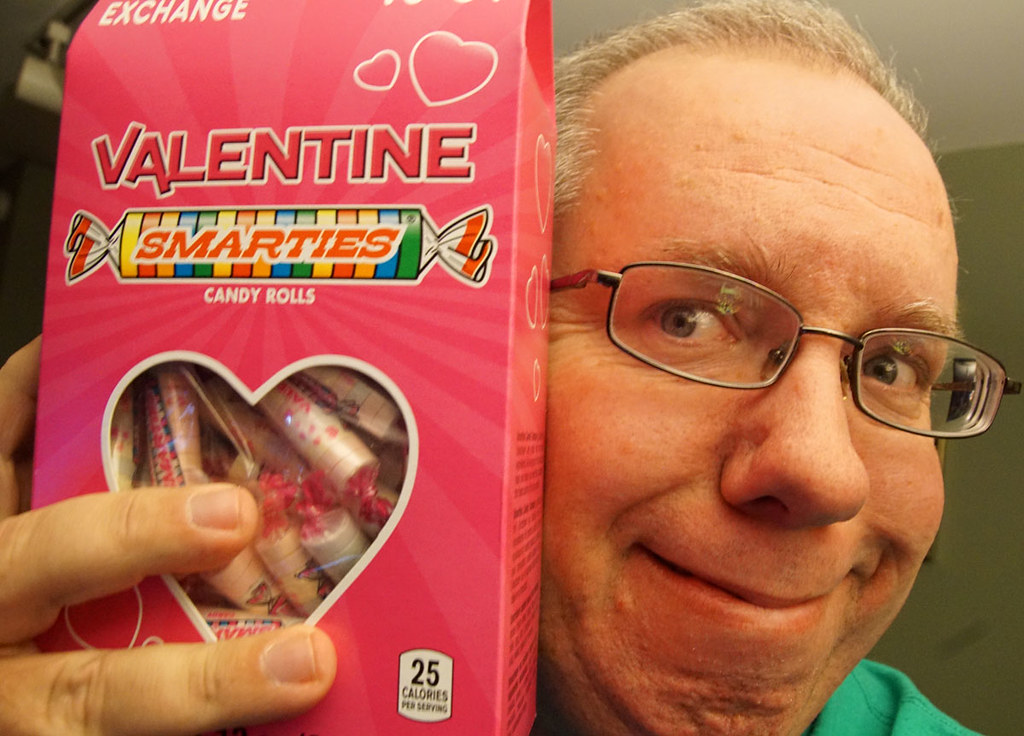In this close-up image, an older Caucasian gentleman with slightly receding, short gray hair and black-rimmed rectangular glasses is prominently featured. He is wearing a turquoise green shirt, visible at his neck and left shoulder. With a cheerful, slightly mischievous smile, he holds a large pink box of Smarties near his face. The box, which he handles with his right hand, showcases a heart-shaped clear cellophane cutout through which the multi-pack of round, colorful Smarties candies can be seen. The words "Valentine Smarties" are boldly printed on the box, accompanied by an illustration of the candies in their distinct wrappers. Additionally, "Candy Rolls" is written in white letters below the illustration, and a small placard at the bottom right of the box states "25 calories per serving" in black lettering. The backdrop suggests a typical indoor setting, adding to the spontaneous and light-hearted nature of the photograph.